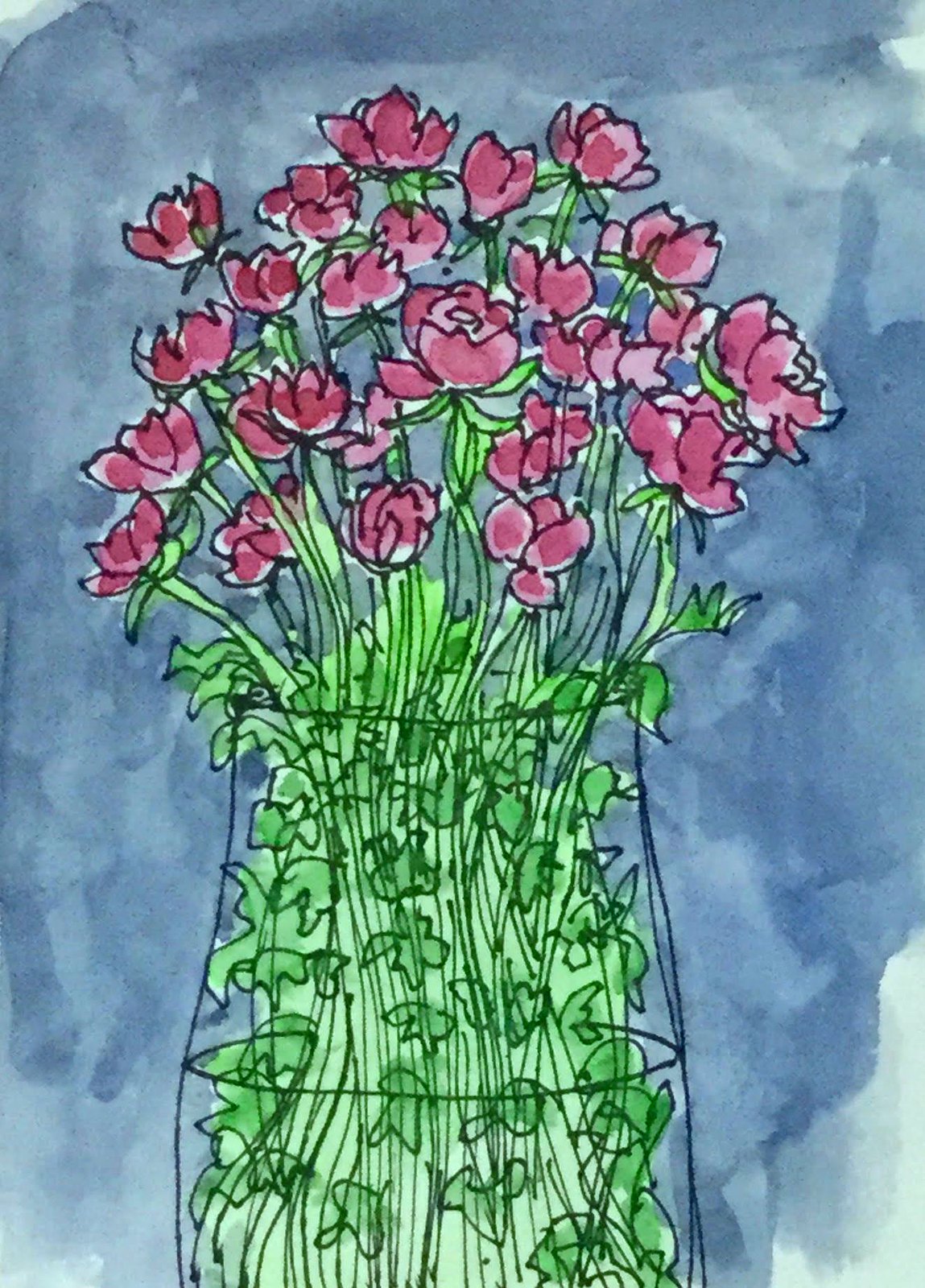This photograph captures a meticulously hand-drawn illustration, featuring a dynamic blend of dark and light blue hues that form a somewhat abstract, blobby background. In the foreground stands a transparent vase, sharply defined with black outlines. Inside the vase, a lush arrangement of leafy green stems, intricately detailed in both dark and light green shades, fills the space with vitality. Atop these stems, a bouquet of exquisite flowers blooms, displaying soft gradients of mauve, light pink, and purple, all delicately outlined in black. The individual petals of the flowers are clearly distinguishable, adding to the overall crisp and clear quality of the image. Notably, the background colors exhibit a subtle bleeding effect, enhancing the artistic depth and texture of the composition.